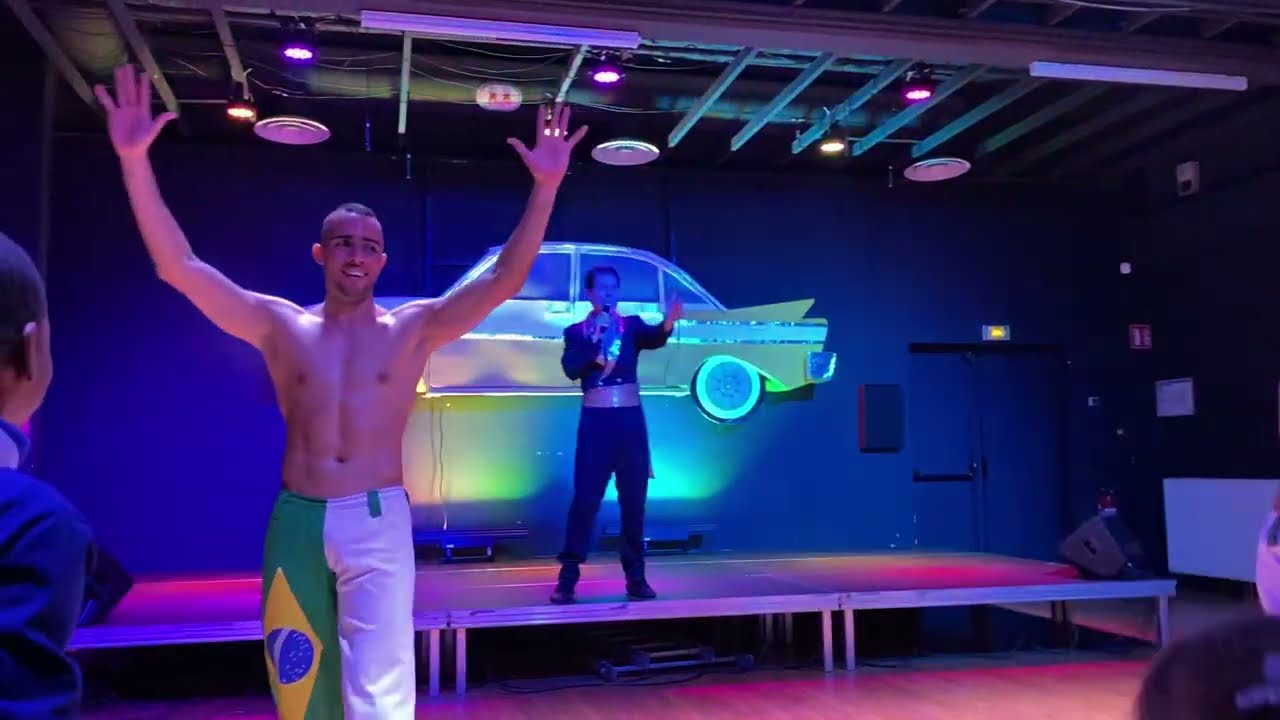In this vibrant and neon-lit image, two primary figures dominate the scene. The room is bathed in hues of purple, pink, and other neon colors, giving it an almost black-light effect. In the foreground on the left, a shirtless young man with an expressive smile stands with his arms raised. His pants are striking, split between white on the left and green with the Brazilian flag on the right. Behind him, elevated slightly on a platform that resembles a ping pong table, stands another man dressed in a black outfit. He holds a microphone in his right hand, raising his left hand as if in mid-speech. To the background, a large, retro-looking car sign with silver and yellow details adds to the nostalgic ambiance. Several other people are partially visible around the periphery, particularly to the bottom right and left of the image.